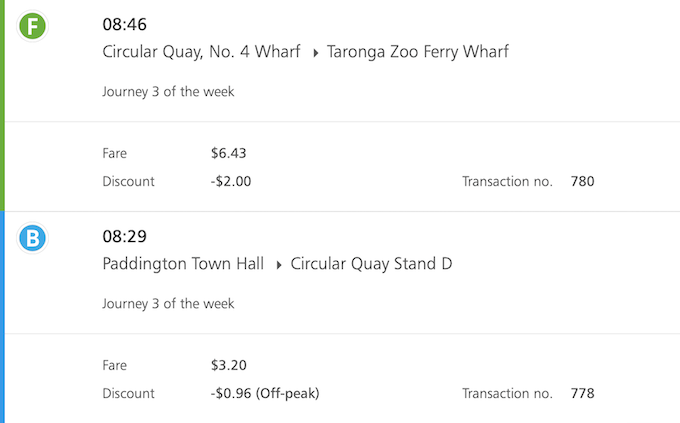**Description of the Image:**

The image appears to detail records of transportation transactions, possibly related to public transit or a bike-sharing service in Sydney. The document prominently features a heading at the top that reads, "Circular Quay No. 4 Wharf," indicating a connection to Taronga Zoo Ferry Wharf 2. 

Here are the notable features and details observed:

- **Date and Time:** The timestamp provided is "46 a.m.," although the exact hours and minutes seem to be unclear or potentially a typographic error.
- **Visual Elements:**
  - A green vertical line runs along the left side of the document from top to bottom.
  - A blue circle containing a white "B" emblem is present.
  
- **Transaction Details:**
  1. **Journey Record 1:** 
     - Noted as the third journey of the week.
     - Originating from Circular Quay No. 4 Wharf to an unspecified location.
     - Fare: $6.43
     - Discount: -$2.00
     - Transaction Number: 780
     
  2. **Journey Record 2:** 
     - Accompanied by a blue line and a "B" symbol.
     - Route: From Paddington Town Hall to Circular Quay Stand D.
     - Fare: $3.20
     - Discount: $0.96 (off-peak fare)
     - Transaction Number: 778
     
Assumptions suggest these might be records of using public transport or potentially for hiring a vehicle like a tuk-tuk or an electric bicycle. The presence of discount details, varying transaction numbers, and distinct journey descriptions support this inference.